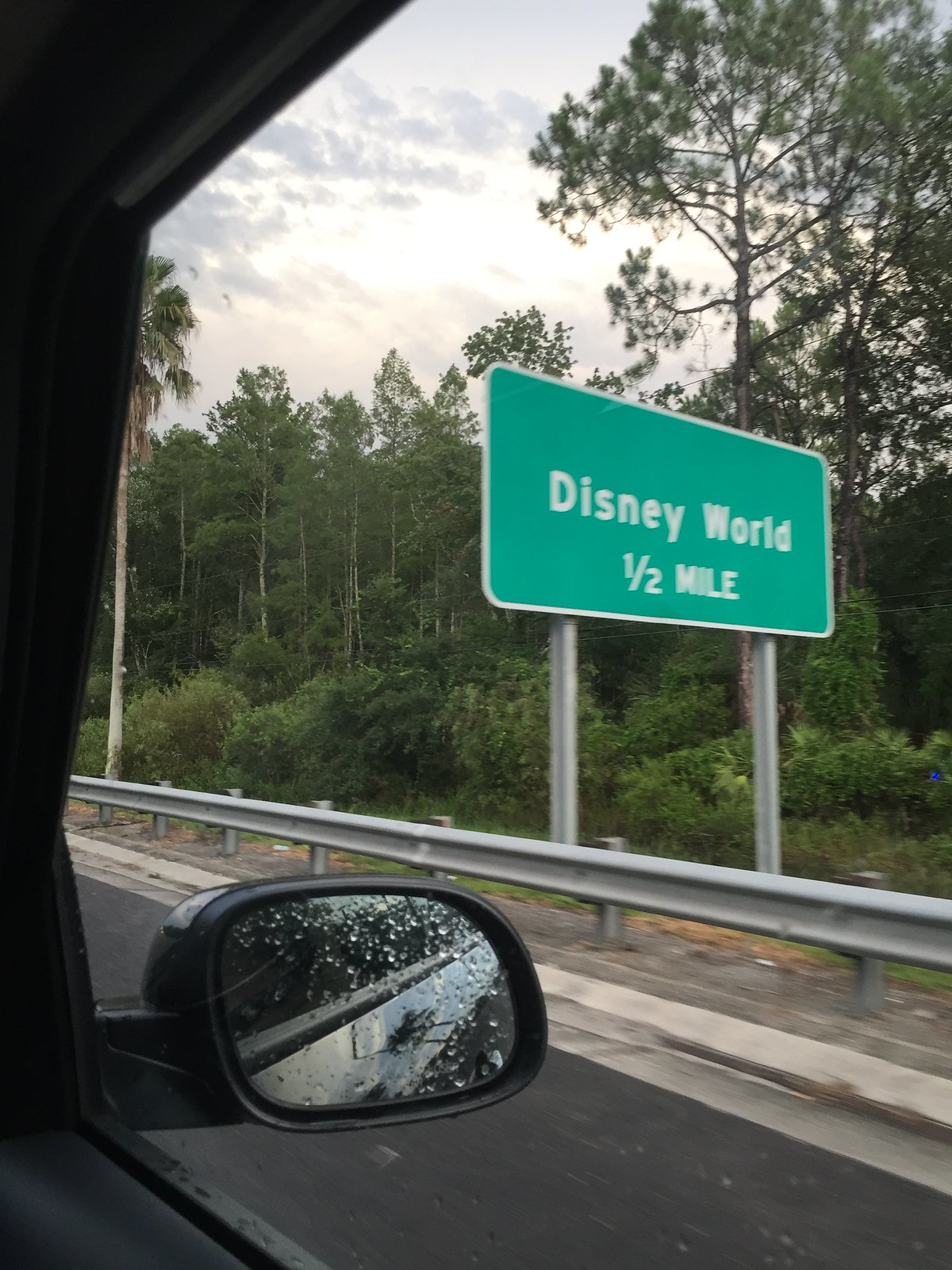This photograph captures a roadside scene featuring a green directional sign indicating that Disney World is a half mile away. The sign is mounted behind a silver guardrail on the right-hand side of the roadway. The sign itself has "Disney World" written in standard upper and lower case letters, while "1/2 MILE" is displayed in all capital letters. The sky is partly cloudy, suggesting an overcast day when the photo was taken.

In the image's foreground, part of a black vehicle is visible, including the passenger side mirror and the edge of the door, indicating that the photo was taken from inside the vehicle on the passenger side. To the far right of the sign, there is dense, overgrown vegetation and tall trees adding a touch of natural scenery to the image.